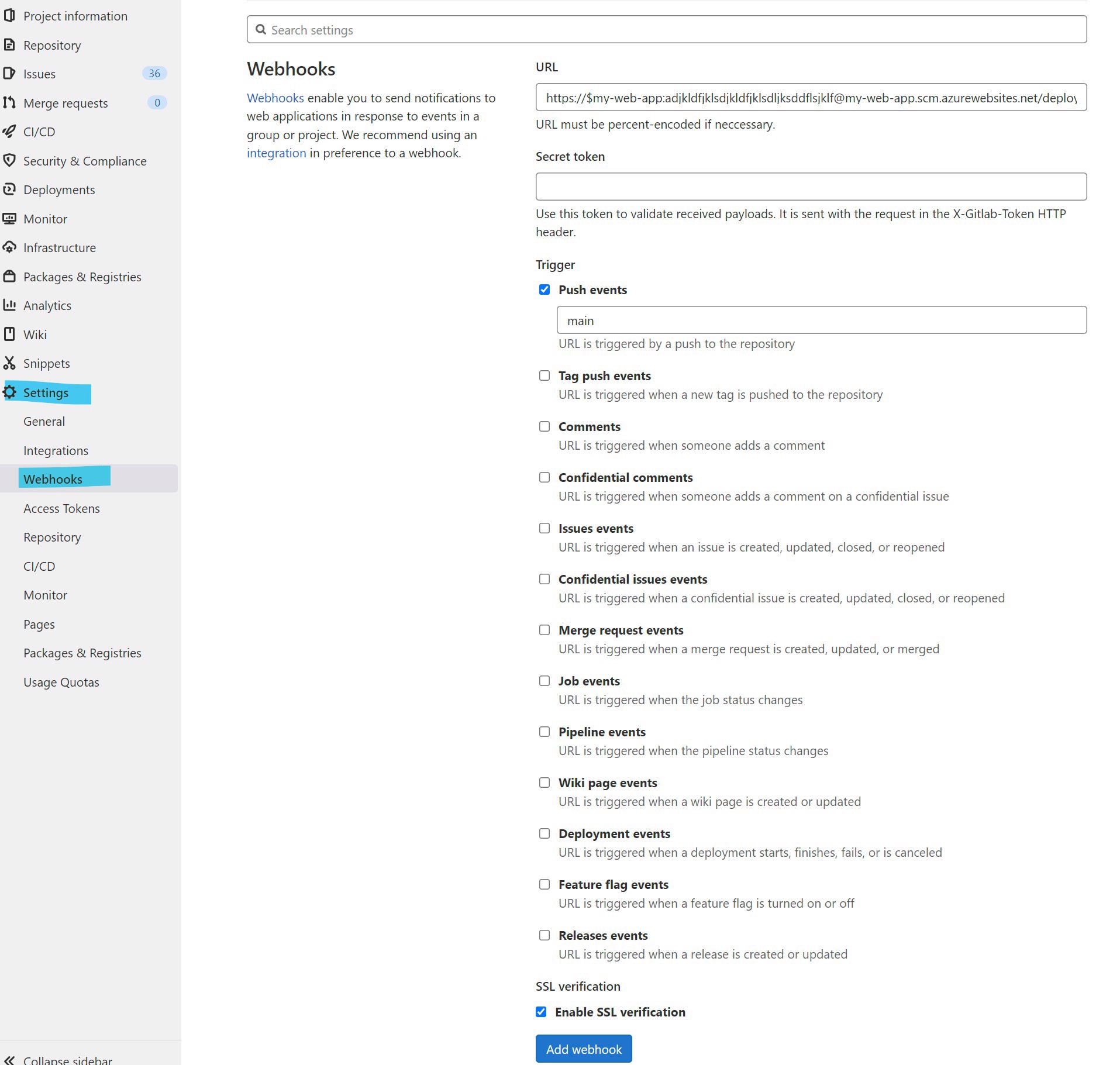**Detailed Caption:**

This image depicts a webpage's search settings interface, specifically focusing on webhooks configuration. At the top, a header clearly states "Search Settings," followed by a section about "Webhooks." The introductory text explains that webhooks enable the transmission of notifications to web applications in response to specific events within a group or project, suggesting the use of integrations over webhooks for better efficiency.

A URL input field is provided, indicating that URLs must be properly encoded if necessary. Below this, there is a "Secret Token" box containing a directive to use the token for validating received payloads, which should be sent with the request in the `X-Gitlab-Token` HTTP header.

The page includes various options organized into boxes:
- **Trigger Options:** Includes checkboxes for events like push events (with "main" specified), tag push events, comments, confidential comments, issue events, confidential issue events, merge request events, job events, pipeline events, wiki page events, development events, feature flag events, and release events.

An "SSL Verification" section is present, with an option to enable SSL verification. This option is currently enabled, as indicated by a checked blue checkmark. 

At the bottom of the webhook settings area, a prominent blue button labeled "Add Webhook" is displayed, indicating the final step to save or apply the webhook configuration.

The overall design of the page is predominantly white, with a side menu and various other options presented on a gray background. The layout and elements reflect a typical web application interface, structured for easy navigation and use.